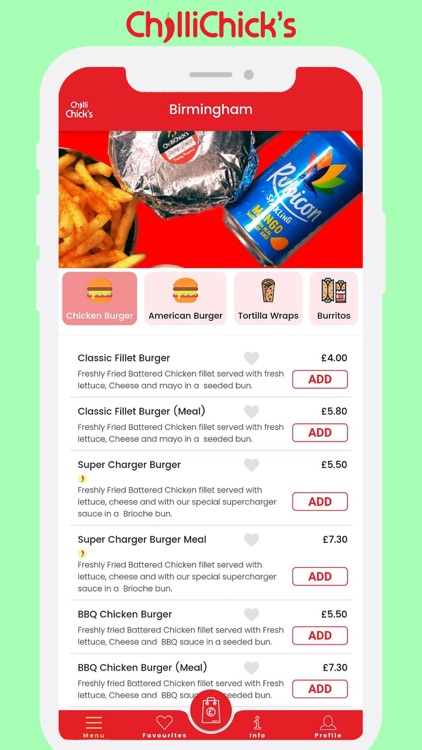The image showcases the interface of the "Chili Chicks" app, which is displayed on a white smartphone. The app's header is vibrant red and prominently features the text "Chili Chicks Birmingham." Below this, there is a mouth-watering photograph displaying crispy fries, a burger wrapped in foil, and a cup of Coca-Cola. Adding to the visual appeal, cartoon-style illustrations depict various food items such as chicken burgers, American burgers, tortilla wraps, and burritos.

The menu segment is comprehensive, listing the following items along with their prices:
- Khalid Classic Fillet Burger: €4.00 
- Classic Fillet Burger Meal: €5.80
- Supercharger Burger: €5.50
- Supercharger Burger Meal: €7.30
- BBQ Chicken Burger: €5.50
- BBQ Chicken Burger Meal: €7.30

At the bottom of the app screen, navigational options are clearly labeled as "Menu," "Favorites," "Info," and "Profile."